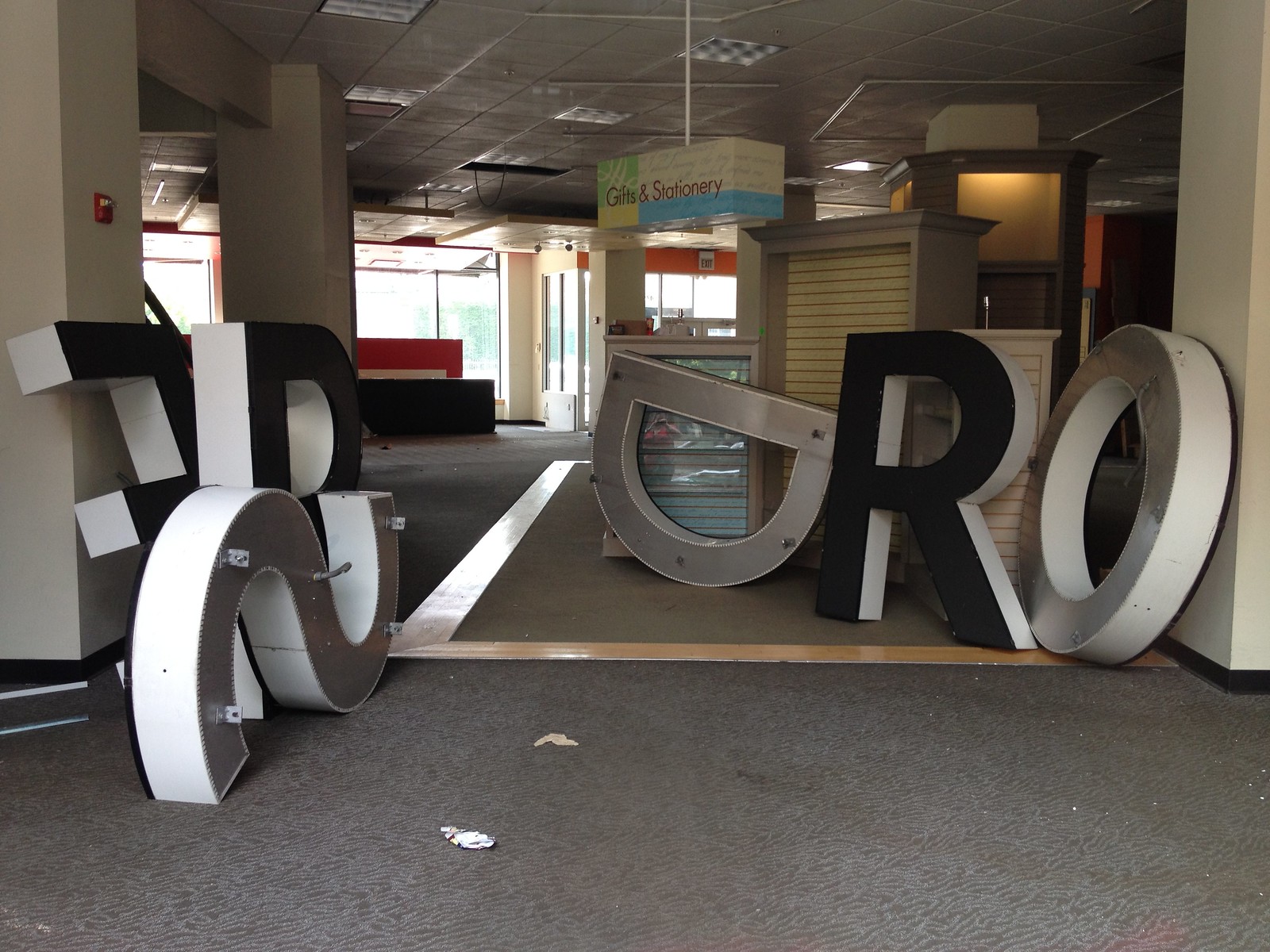The image depicts the interior of a closed store, likely a department store or possibly a FedEx or UPS location. The ambiance is dim, with pillars made of drywall and a somewhat dirty, gray carpeted floor. Dominating the scene are large, disused letters—E, S, D, R, O, and P—formerly part of an exterior sign, now resting haphazardly on the carpet. In the background, furniture is stacked behind the letters, and empty cabinets and shelves can be seen. Hanging prominently from the ceiling at the top center is a 3D rectangular sign in green, yellow, and blue, which reads "Gifts and Stationery," a relic from when the business was operational.